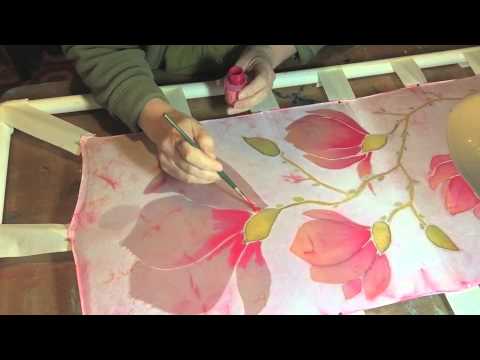The image is a high-angle, full-color shot capturing a person, mostly out of frame, sitting at a work table, engaged in painting a flower design on a long, rectangular fabric piece, about two feet wide and four feet long. The primary visible elements are the person's hands—right hand wielding a green paintbrush dipped in bright pink fabric paint and left hand holding a small paint bottle. The person, donning a green sweater, is meticulously painting large flowers on the white fabric. Each flower features a gradient detail, with darker pink at the petal bases transitioning to lighter pink towards the tips. The flowers, three in total, are connected by green stems that stretch from top to bottom of the fabric. The workspace is well-lit, highlighting the vivid colors of the artwork and the details of the fabrication process, which occurs on what appears to be a wooden table. The fabric seems to be supported on some kind of wooden frame or nailed support. The scene is clearly part of an artistic endeavor, reflecting a serene and focused atmosphere.